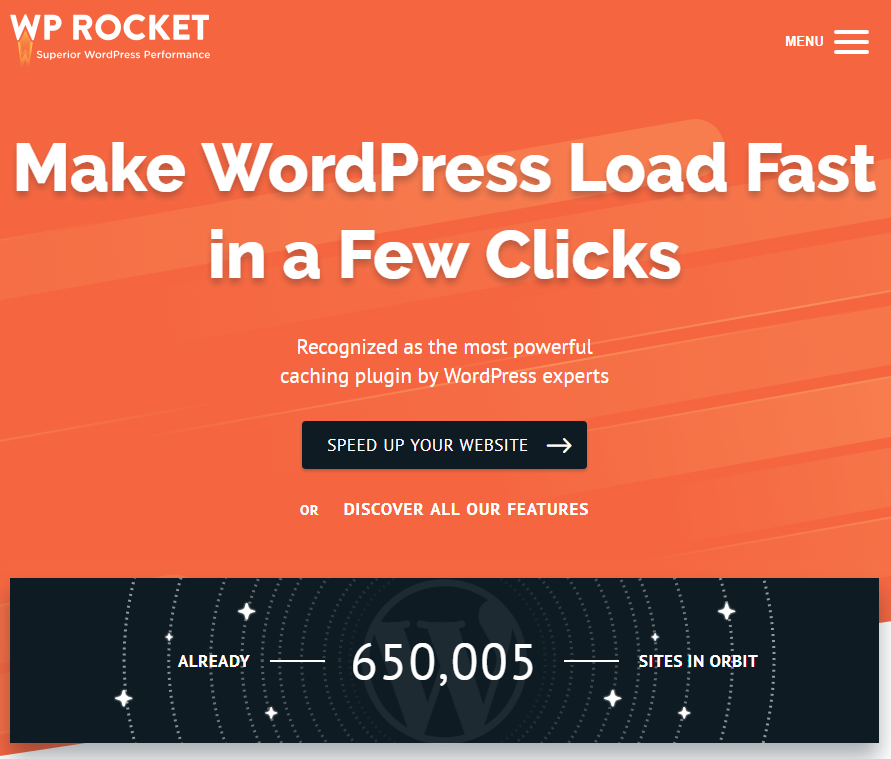"This promotional image for WP Rocket highlights Superior WordPress Performance. Dominated by an orange background, the layout features a stacked menu icon labeled 'Menu' on the right side. The main message, 'Make WordPress load fast in a few clicks,' stands out in large white font. Below, text declares WP Rocket as 'recognized as the most powerful caching plugin by WordPress experts.' A prominent black button with white text and a right-pointing arrow reads 'Speed up your website,' followed by an invitation to 'discover all of our features' in smaller white text. The bottom strip of the image is black, displaying the text 'Ready, 6,505 sites in orbit' alongside an illustration of Earth surrounded by orbiting dots, symbolizing the websites enhanced by WP Rocket. The color palette consists mainly of orange, black, white, and possibly gray."